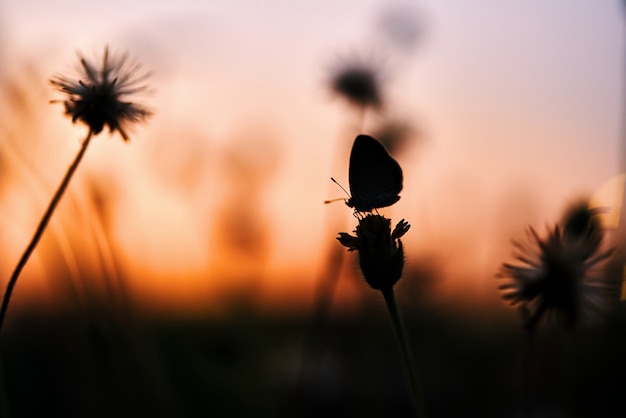An outdoor scene at dusk captures a striking sky transitioning from a deep, light purple at the top to a warm, glowing orange at the horizon, signaling the sun's last light. The foreground presents the silhouettes of various plants, prominently featuring potential dandelions with long stems and small, circular heads, poised to disperse seeds. On the far right, a dandelion-like plant stands out with long, thin petals. At the center, a taller plant is crowned by the delicate form of a butterfly or moth, wings upright and antennas visible. The ground is enveloped in darkness, with the obscured shapes of grass or wheat adding texture to the background, completing this tranquil yet richly detailed sunset tableau.